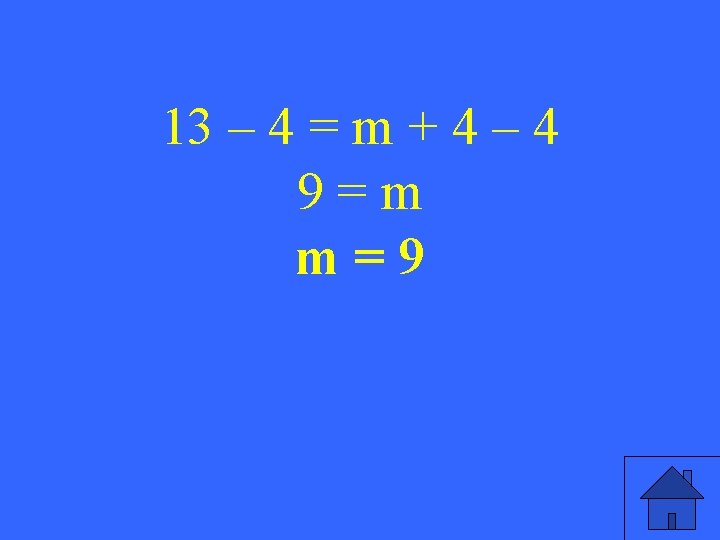This image features a royal-to-light blue rectangle, wider than it is tall, which appears to be part of an educational PowerPoint slide. Against the blue background, centered towards the upper portion of the rectangle, are three lines of yellow text depicting a math problem. The first line reads "13 - 4 = M + 4 - 4," the second line centers below it stating "9 = M," and the third line reads "M = 9," positioned just above the midpoint of the image, leaving the bottom half predominantly blue. In the bottom right corner, there is a small, crudely drawn house logo. The house consists of a dark gray triangle roof, with a small chimney on the right side, a rectangular blue-gray body, and a thin black rectangular door, all outlined within a black square frame that lacks its bottom and right sides. The logo is simplistic and geometric, juxtaposed against the educational content, emphasizing the potential classroom setting of the slide. The overall color palette includes different shades of blue, black, and yellow.